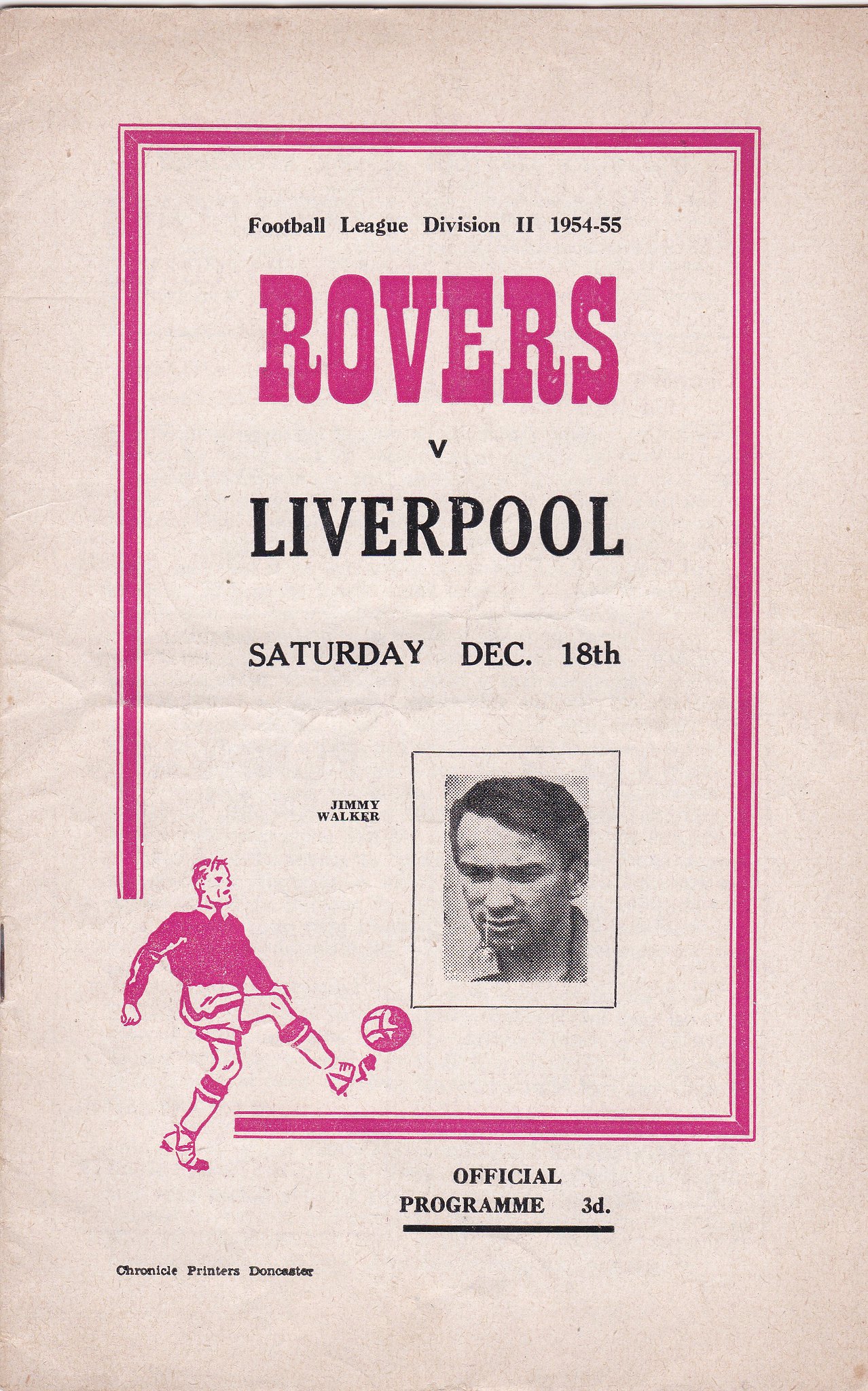The image is an old sports program printed on a light pink stock with predominantly darker pink text. It features a black and white photograph of a man labeled as Jimmy Walker, positioned towards the middle of the program. The event is a match between Rovers and Liverpool, occurring on Saturday, December 18th, as part of the Football League Division 2 for the 1954-1955 season. In the lower right-hand corner, there is a drawing of a soccer player kicking a ball, also in pink. The text is framed with a pink border, enhancing its vintage appeal.